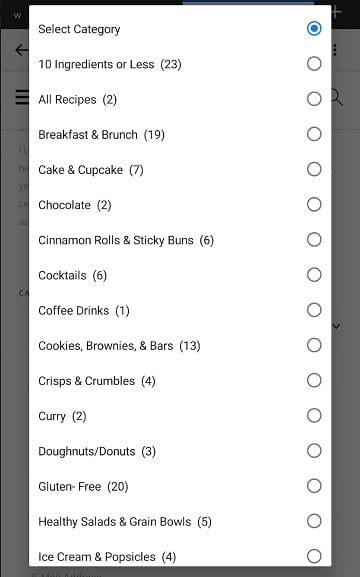The image features a comprehensive list of food categories set against a diverse background. The central portion of the image is dominated by a white background, while the left, right, and very bottom edges are bordered by a narrow gray background. The top two corners of the image feature a black background. 

At the right end of each category item, there is a small circle, used for selection, with only the top category, labeled "Select category," highlighted and selected in blue. The categories are listed from top to bottom as follows:

1. Select category
2. 10 Ingredients or Less
3. All Recipes
4. Breakfast and Brunch
5. Cake and Cupcake
6. Chocolate
7. Cinnamon Rolls and Sticky Buns
8. Cocktails
9. Coffee Drinks
10. Cookies, Brownies, and Bars
11. Crisps and Crumbles
12. Curry
13. Donuts/Donuts
14. Gluten-Free
15. Healthy Salads and Green Bowls
16. Ice Cream and Popsicles

Each category has a corresponding number enclosed in parentheses positioned to the right, indicating the number of items or recipes available in that category. The image provides an organized and visually sorted interface for selecting different types of food-related content.